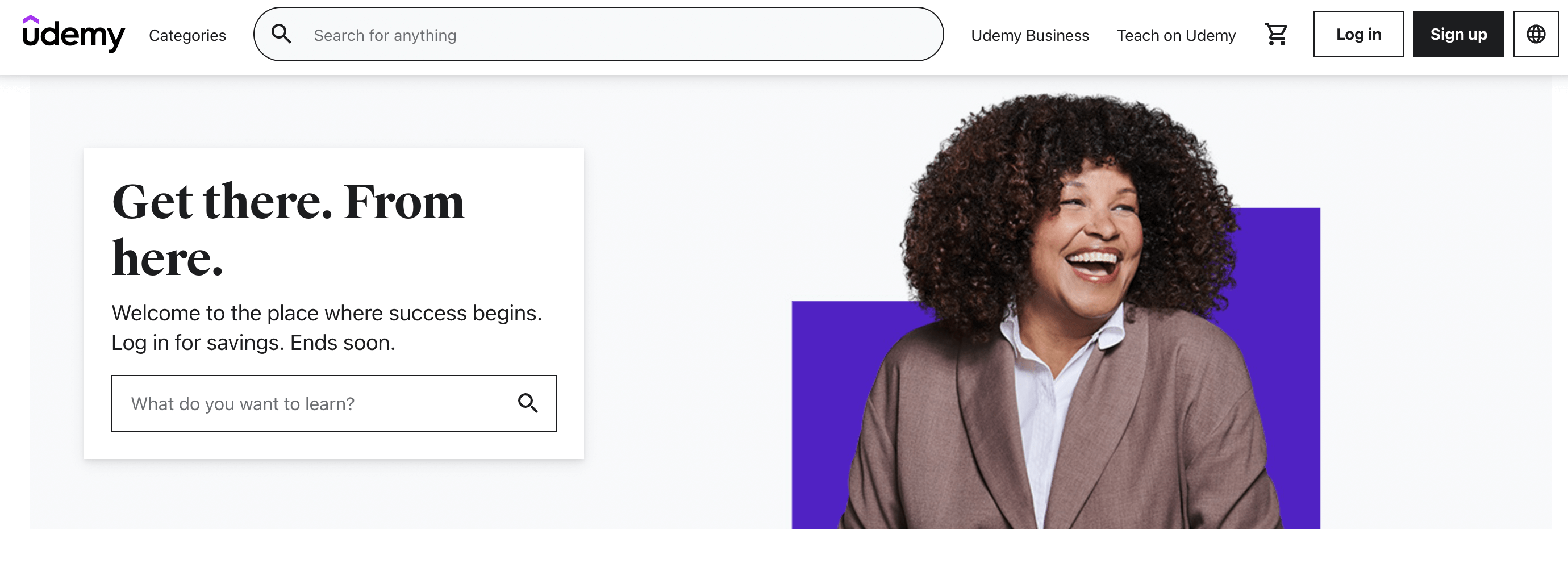This image is an advertisement for Udemy, prominently showcasing the Udemy website interface. At the top, the word "Udemy" is displayed in bold black letters, accompanied by a stylized 'U' with a purple, almost triangular symbol above it. To the right of the logo, the section labeled "Categories" is visible. Underneath is a large search bar with a magnifying glass icon and the placeholder text, "Search for Anything." 

Adjacent to the search bar are several menu options: "Udemy Business," "Teach on Udemy," and icons for a shopping cart, a login button with a white background and black lettering, and a sign-up button featuring a black background with white lettering. There's also a globe-like symbol represented in black with intersecting lines, possibly indicating language or location settings.

Below these elements, a white box with black text proclaims, "Get There From Here, Welcome to the Place Where Success Begins, Login for Savings, End Soon." Another search bar follows, asking "What Do You Want to Learn?” with another magnifying glass icon to the right.

To the right of these interface details is a vibrant image of a woman with beautiful, bouncy brown curls. She is smiling broadly while wearing a brown blazer over a white collared shirt and brownish lipstick. The background behind her is a striking bluish-purple, providing a vivid backdrop to her joyful expression.